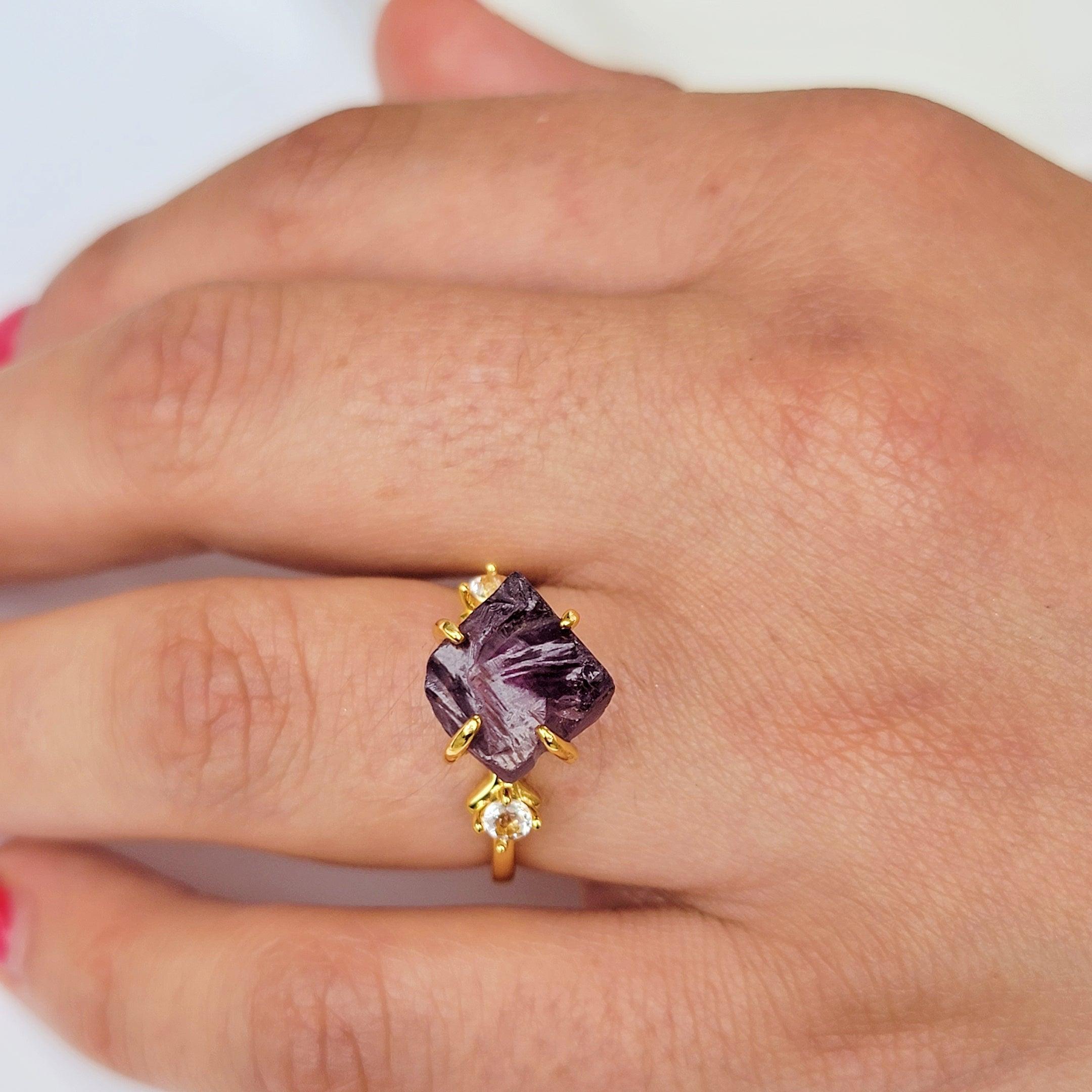The image showcases a detailed close-up of a Caucasian female's left hand with a medium skin tone, focusing on her left ring finger, which bears a striking gold ring. The ring features a prominent purple gemstone, imbuing rich amethyst-like hues with various shades of white reflecting as light catches its jagged contours. This central stone, held securely by four gold prongs, is flanked by small round stones—likely diamonds or cubic zirconia—set in the same gold band. Her fingernails are painted in a carnation-colored pink polish, notably on the forefinger and pinky. The hand's knuckles exhibit a reddish-pink tinge, and the overall image is a well-composed square, with the foreground in sharp focus while the background is slightly blurred for depth.